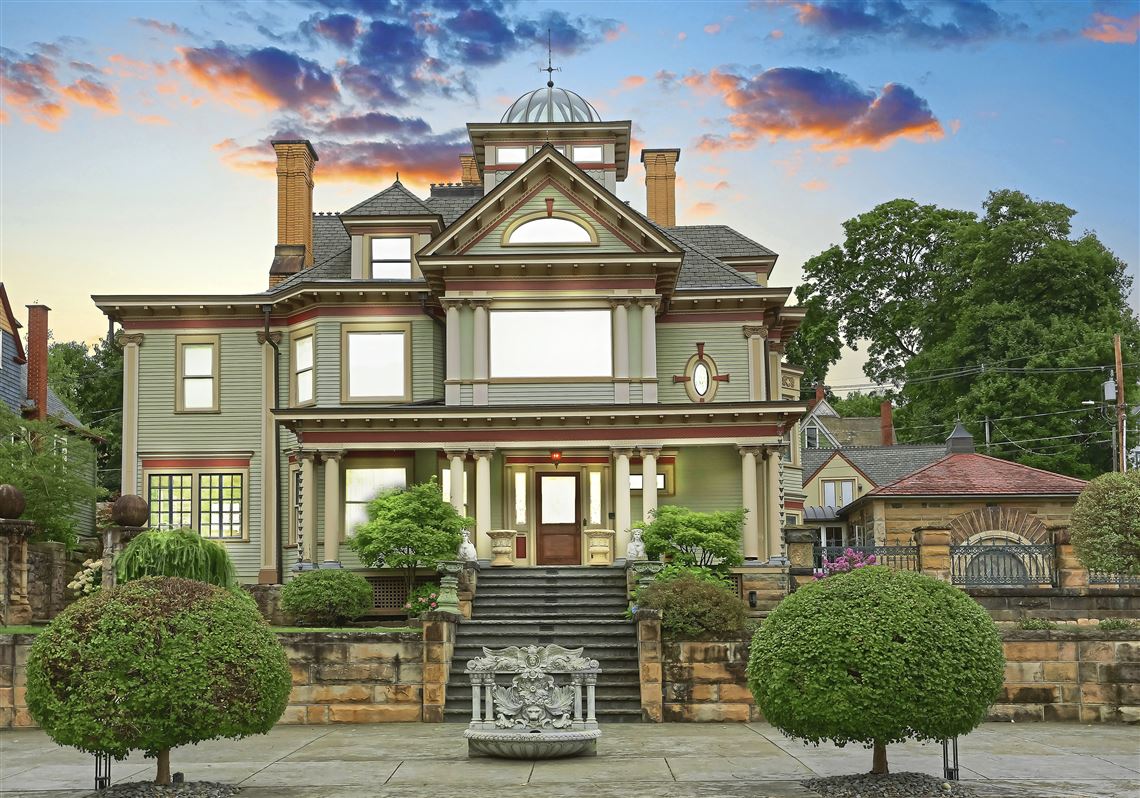This photograph depicts a striking Victorian-style home with contemporary updates, enhanced to appear almost like a painting. The two-story house, possibly appearing to be taller due to its elevated position, has a greenish hue that might also seem pale blue or gray depending on the lighting, which is around dusk, adding a magical quality to the scene. The grand entrance is made of meticulously arranged stone blocks and features two impressive flights of stairs, elevating the house approximately 15 feet above the expansive, square, gray-green cement courtyard. Decorated with circular bushes and a decorative stone fountain, the courtyard adds to the home's grandeur. There is also a small porch area supported by elegant white marble columns, which are echoed on the second floor, and a warm brown front door. The house boasts detailed wood sidings, two large chimneys, and a distinctive clear dome on the roof, further enhancing its Victorian charm. The setting sun illuminates a few clouds in the sky behind the house, rounding out this image of a house that combines vintage elegance with modern design touches.